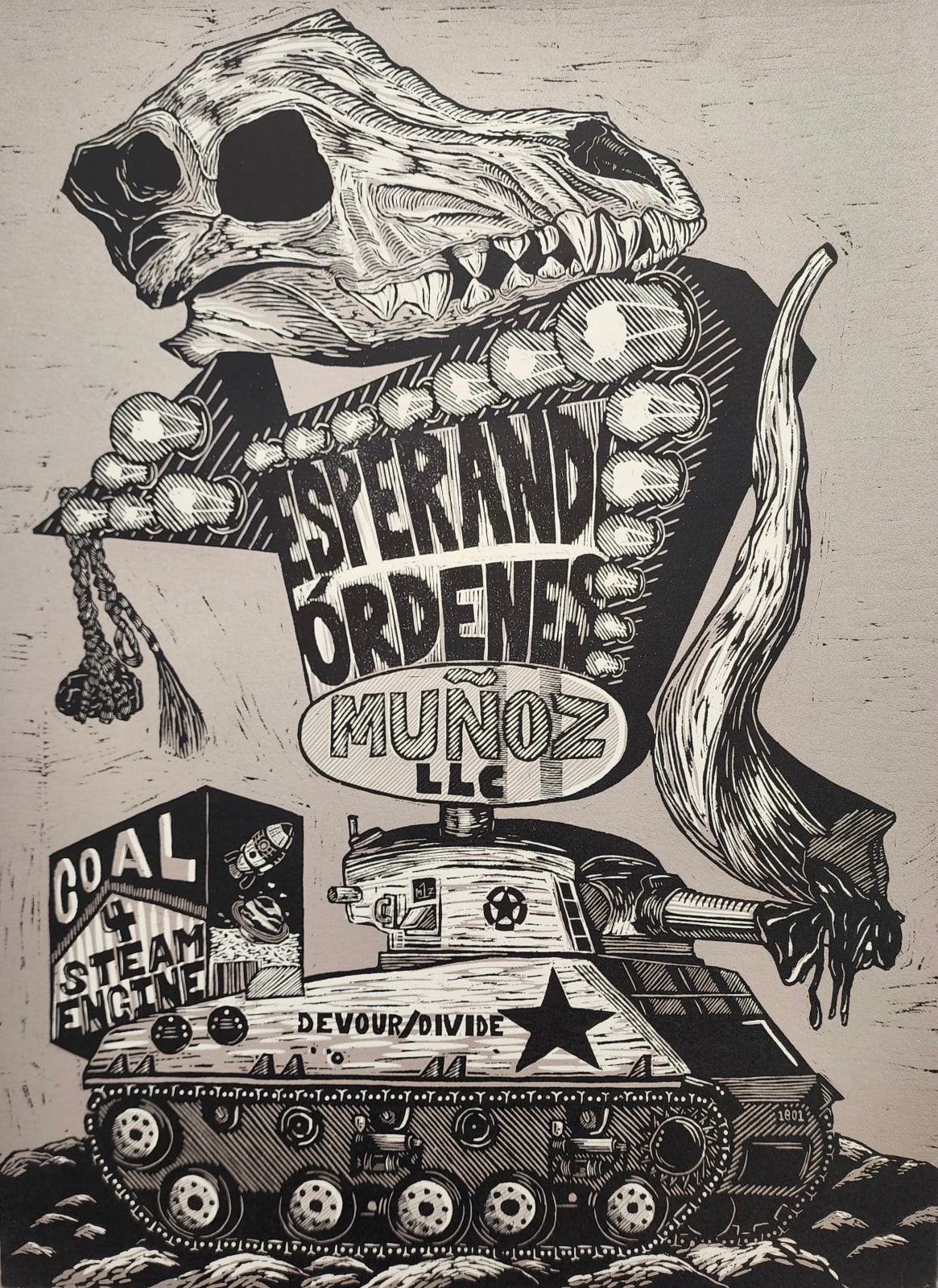This detailed pen and ink illustration, set against a beige background, portrays a military tank moving over uneven, rocky ground. The tank bears the inscription "Devour/Divide" alongside a prominent dark star. On top of the tank, a retro, Broadway-style neon marquee sign with light bulbs and an arrow pointing left reads "Esperando Ordonez Munoz LLC." A large, imposing skull with sharp teeth sits atop this sign, adding an element of macabre intrigue. To the left, there's a box labeled "Goal 4 Steam Engine," depicting the planet Saturn and a rocket ship. The artwork is rendered in black and white with extensive shading and cross-hatching, highlighting its grunge style.